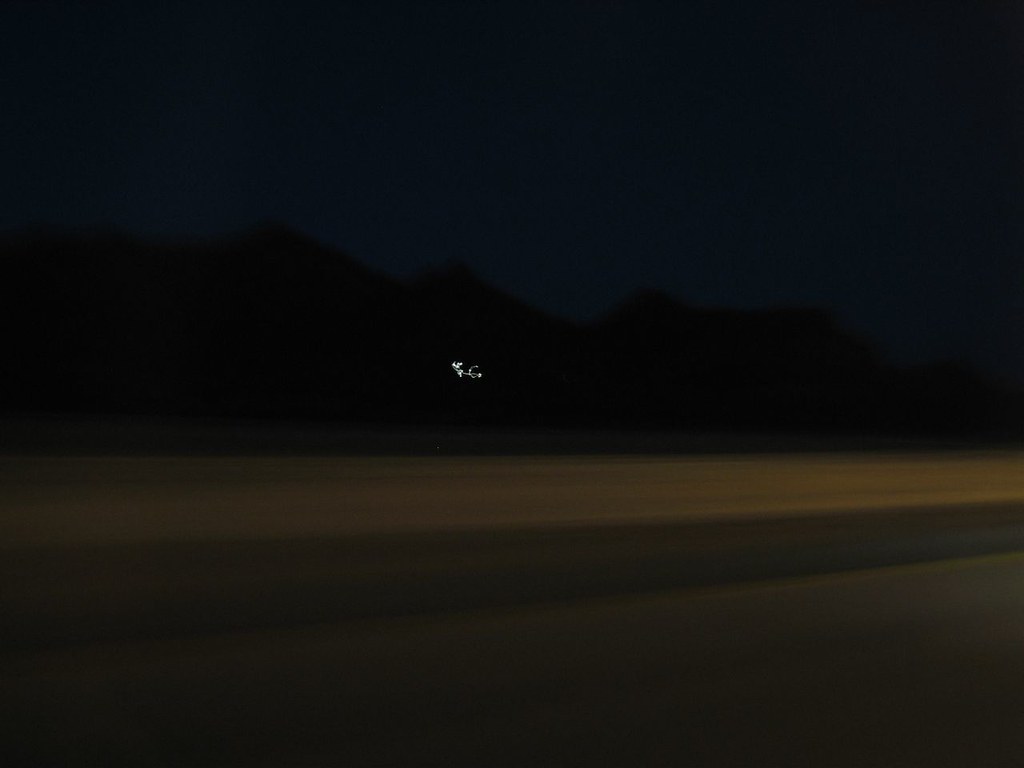The image is a horizontal rectangle dominated by darkness and subtle, indistinct features suggestive of a night scene. The upper half of the image is almost entirely black, with just a hint of dark blue or off-black adding a slight variation in the otherwise uniform darkness. This vast, dark expanse stretches from left to right, reaching down about one-third of the image before it meets a faint silhouette of a mountain range. The mountain range is a shadowy presence, with subtle variations in height, appearing somewhat jagged and flattened in places. 

In the center of the image, amidst the blackness of the mountains, there is a very small, indistinct white figure, appearing almost like a distant, glowing object or perhaps even a tiny kite. This white figure is extremely tiny and hard to distinguish due to the image's blurry and dark nature.

Below the mountains, a lighter, yet still dark, tan area emerges, creating a vague strip that blends into a brownish hue towards the very bottom of the image. This bottom section comprises a series of indistinct, fuzzy stripes—a thin gray line, followed by a thicker brown line, and another thinner gray line, giving a layered appearance. The overall effect is a hazy and blurry view, with the lighter sections providing a slight contrast against the dominating darkness.